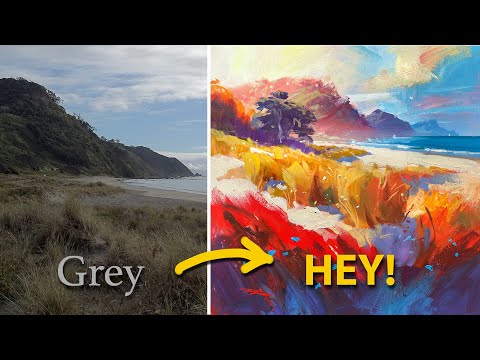This horizontal rectangle image features two side-by-side renditions of a coastal landscape, surrounded by black bars on the top and bottom. On the left, there's a realistic photograph that is labeled "gray," capturing a muted, dimly lit scene with a hill or mountain in the background, beige-ish dry grass in the foreground, sand, and a stretch of water under a blue, cloudy sky. Positioned above the word "gray" is a yellow arrow pointing to the right side of the image. The right side presents an artfully dramatized, colorful painting of the same scene. Here, the grass is vividly rendered in red, white, and yellow hues, the sand appears yellow, and the water a bright aqua blue. The sky is filled with red light, casting purplish-yellow tones on the mountain. In yellow font, the word "hay!" adds a lively touch. The vibrant colors and thick brush strokes give the image on the right much more depth and dramatic appeal.